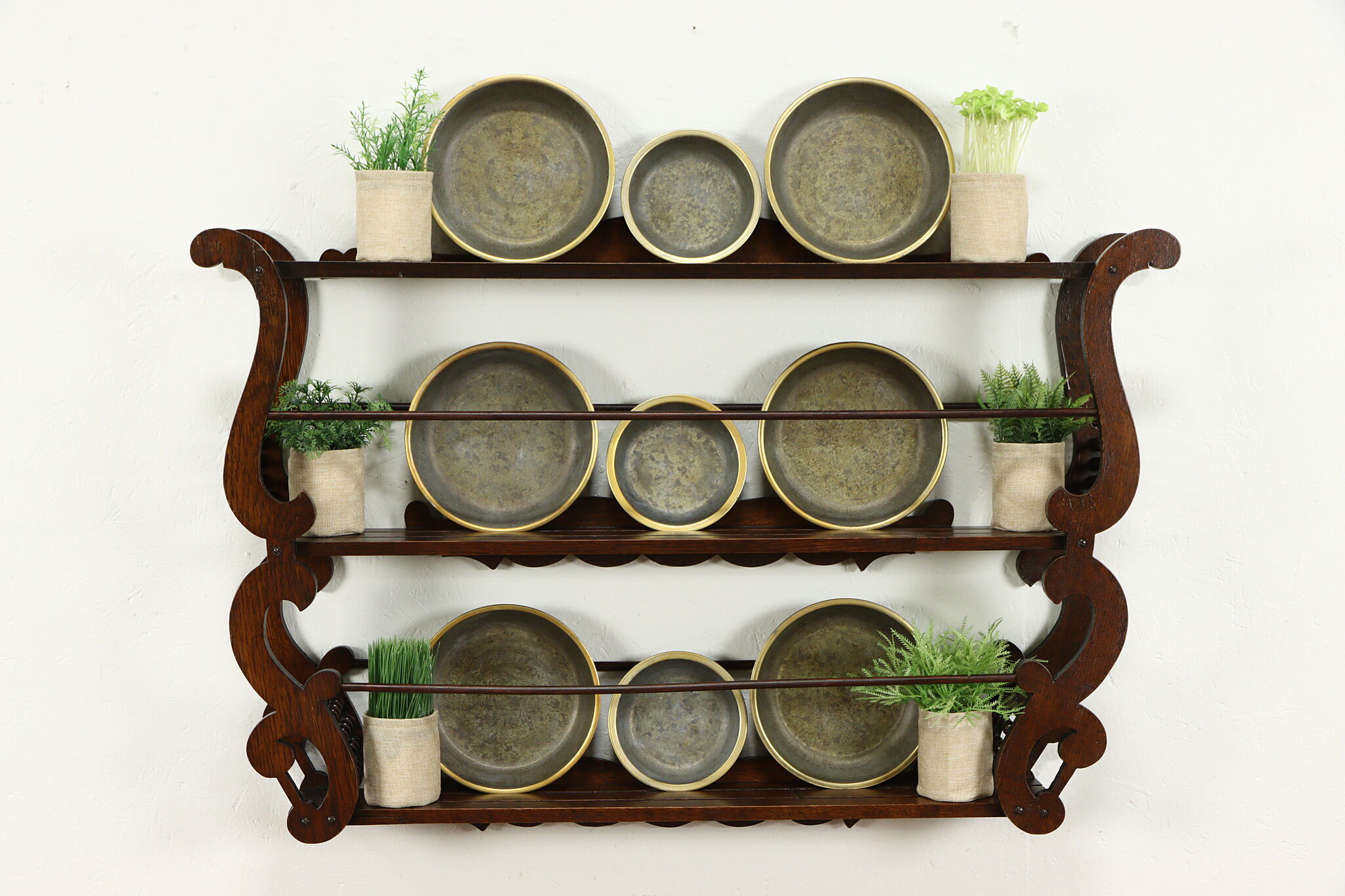This image showcases a decorative wall-mounted shelf set crafted from dark brown wood, featuring ornate scrolling details on either end. The shelf spans three levels, each meticulously adorned with a trio of plates, displayed sideways to reveal their intricate design. The composition on each layer includes two large plates on the sides and a smaller plate centered between them. The plates exhibit a striking appearance with a grayish hue and gold trim, the insides displaying a deeper brownish-gold. Flanking each plate arrangement are white ceramic pots containing verdant plants. These plants vary in type, showcasing an array of greenery including grassy plants, leafy sprouts, and ferns. The backdrop is a pristine white wall that highlights the elegance and detail of the shelving unit and its contents.